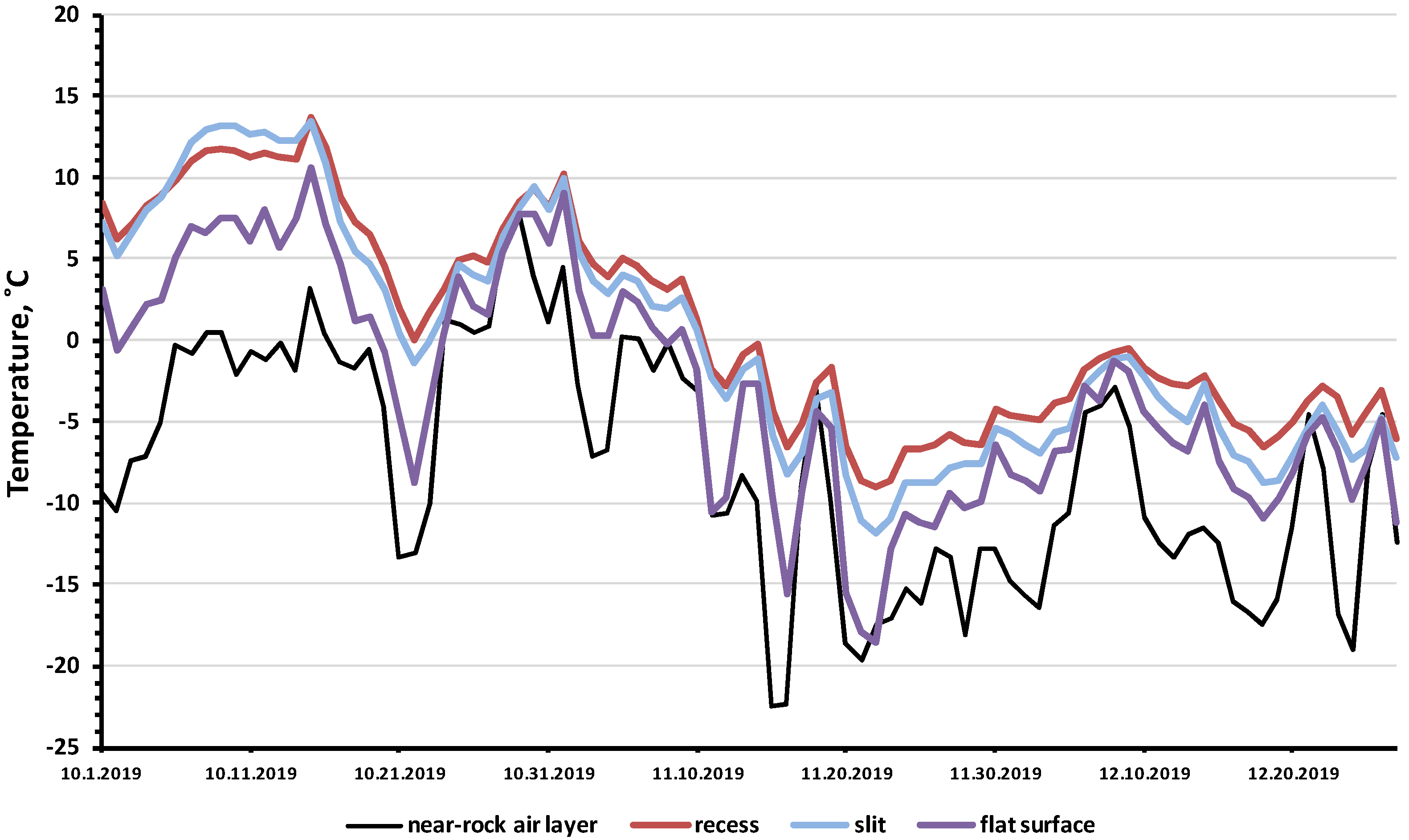This image depicts a detailed line graph on a white background, characterized by horizontal thin gray grid lines and black X and Y axes. The X-axis, which represents dates, starts on the left with 10-1-2019 and progresses through 10-11, 10-21, 10-31, 11-10, 11-20, 11-30, 12-10, and finally to 12-20-2019 on the right. The Y-axis indicates temperature in Celsius, ranging from -25 degrees at the bottom to 20 degrees at the top, marked in increments of five degrees.

The graph features several colored lines each representing different measurements: the black line for the near rock air layer, the red line for recess, the blue line for slit, and the purple line for flat surface, as per the key located below the X-axis. Starting from the left side, these lines display overlapping, jagged paths with several spikes and dips, yet presenting an overall downward trend as the dates advance. The blue line is observed to start at 10 degrees Celsius, dip to -10, rise slightly to -5, and exhibit similar fluctuations to other lines throughout the graph.